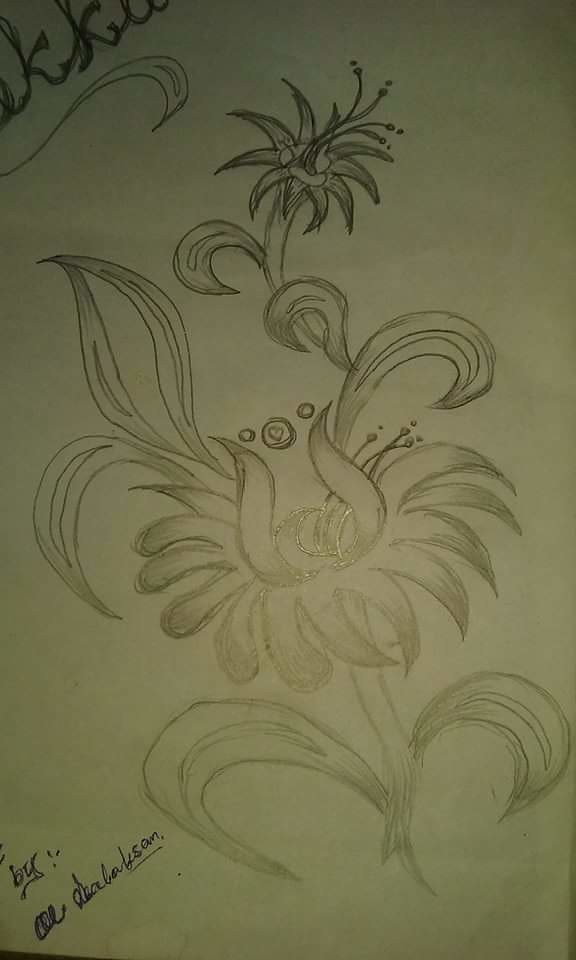The image is a detailed pencil drawing on a white or off-white piece of paper, depicting a stylized flower with intricate details. The central flower resembles a daisy, featuring a short stem with two large leaves extending from its base. The flower’s petals droop downward and include a mix of rounded and pointed shapes. The central part of the flower contains three bubbles, one of which encircles a heart. 

Two long, S-shaped petals curve out from the middle and are pointed at the tips. Additionally, another delicate flower emerges from the right side of the main stem, characterized by triangular petals and elongated, hair-like structures ending in black dots, suggesting pollen. In the upper left corner, a narrow leaf curls elegantly under itself.

The drawing is monochromatic, rendered entirely in pencil, with no added color. Hints of additional elements include bold black symbols or wires drawn in the top left corner, and a signature in cursive at the bottom left, though it remains illegible except for the initials “KK” at the top.